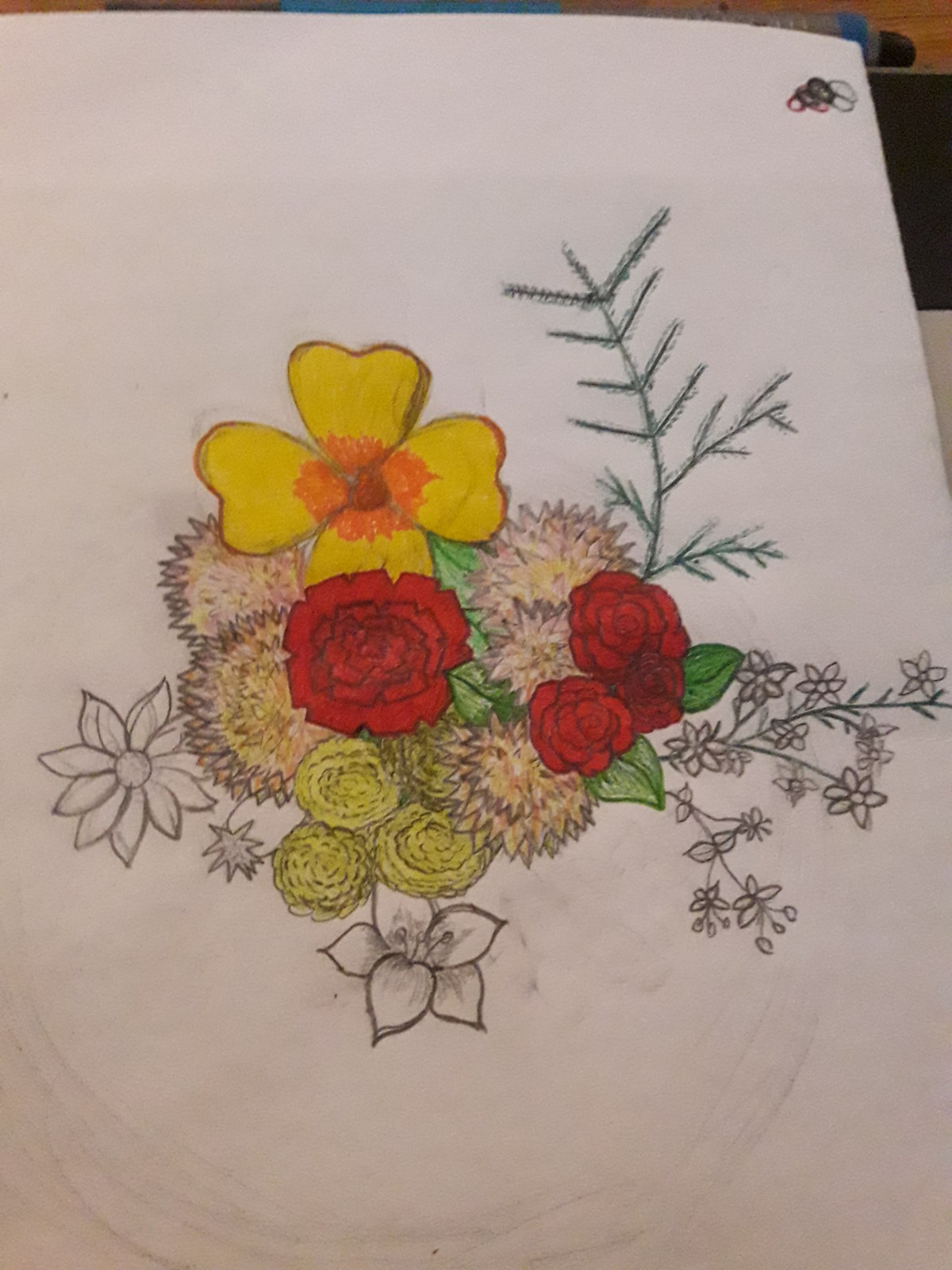This detailed image showcases an elaborately crafted sketchbook drawing of a vibrant and intricately colored floral arrangement. Central to the composition are vivid yellow, orange, red, pink, and green hues that breathe life into flowers positioned meticulously in the middle of the page, with smaller flowers and stems branching out from the central focus. This artistic piece is drawn using pencil and ink, with portions already colored and others still in pencil, creating a dynamic contrast. The arrangement includes a variety of flowers such as roses, daisies, mums, possibly a peony and ranunculus, along with delicate elements like baby's breath. Greenery sprouting from the top adds depth to the arrangement. The artist's skill is evident in the subtle shading and color manipulation, producing a nearly three-dimensional effect. Set against the crisp backdrop of regular white drawing paper, this piece reflects a moment of focused creativity, appearing as though it belongs in an artist’s sketchbook or a casual yet meticulous doodle session, capturing the intricate beauty of flowers in both completed and in-progress forms.